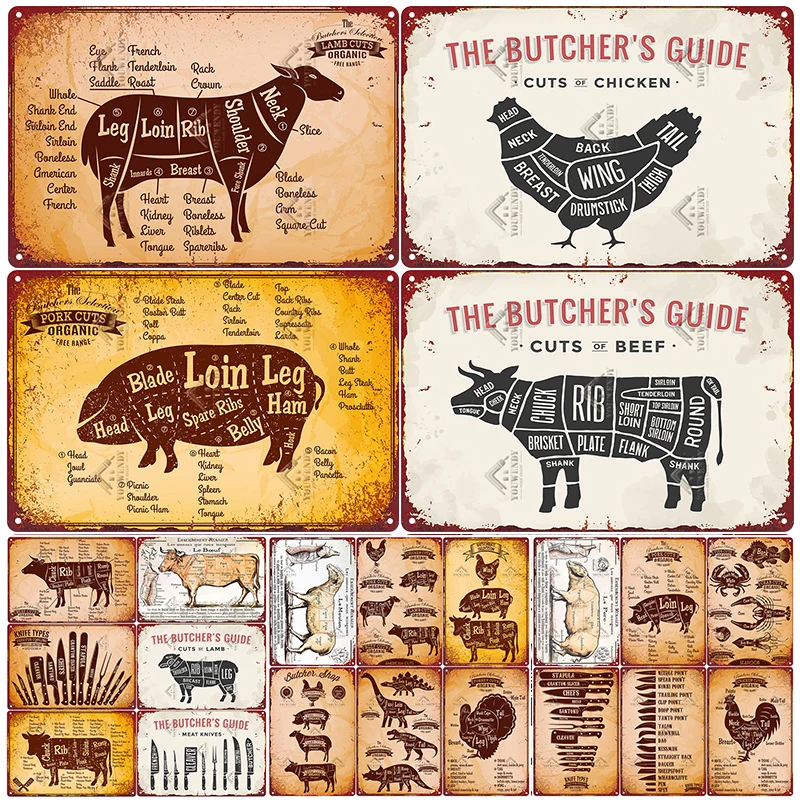The image comprises a detailed collection of butchery diagrams, displayed in a visually cohesive manner. The top two-thirds of the image feature four primary sections, each dedicated to a different animal. 

In the top left corner, there is a diagram of a lamb against a light orange background. The lamb is depicted in a dark red silhouette, with all its parts meticulously labeled. Next to it, in the top right, is a guide labeled "The Butcher's Guide to Cuts of Chicken." This section has a black silhouette of a chicken facing left, set against a white background with a red text header, and its parts are labeled in white text.

The bottom left section is for pork, with a dark orange background and a red silhouette of a pig facing left. This diagram is labeled with orange text, with the inscription "Pork Cuts, Organic, Free Range" at the top left of the section. The bottom right features a guide on beef cuts, showcasing a black silhouette of a bull facing left on a white background. Similar to the chicken guide, it has a header in red text reading "The Butcher's Guide," with "Cuts of Beef" beneath it in black text, and the parts are labeled in white text.

The lower part of the image consists of 18 smaller diagrams and additional posters that replicate various parts of the top sections and introduce new elements like turkeys, dinosaurs, and butchery knives. These smaller images appear as though they could be postcards, each with a distressed, rustic appearance, suggesting they might be found in a butcher’s shop or gift store. The entire composition has a vintage, collage-like aesthetic, tied together by a consistent theme of educating on different cuts of meat from various animals.